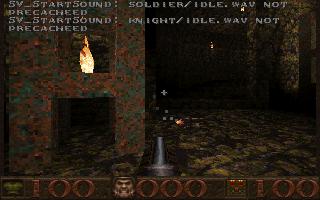This is a small, color screenshot of the classic video game Doom, displayed horizontally. The scene reveals the dark, cavernous interior of a castle-like building, constructed with stone textures. On the left side, there is an architectural element resembling a building with a walkway underneath, depicted in orange, gray, and black marble. The bottom of the screen features a detailed HUD (Heads-Up Display) with a Greek-like ancient face, various numerical values, and circular designs. Specifically, from bottom left to bottom right, is the number 100, followed by an aggressive-looking face, then zeros, another square, and the number 100 again. Flames flicker in the background, adding to the ominous atmosphere. The interface elements and text at the top of the screen indicate the game's state, with lines such as "by start sound soldier/idle.wav not precached" and "5v start sound night/idle.wav not precached." In the foreground, a shotgun is visible, emphasizing the shooter nature of the game. This detailed scene conjures the distinct, nostalgic essence of Doom.